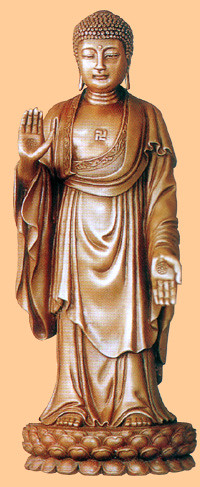The photograph captures an ancient Buddhist statue in great detail, standing upright against a faded orange or tannish pink background. The statue, made of bronze and gold tones, depicts a religious figure adorned with a robe and standing on a platform. The figure's head features a distinctive covering with bumps or ridges, possibly symbolizing hair or a traditional headpiece, and a noticeable dot between the eyes. The statue’s expression is serene and contemplative, with earrings adorning its ears. One hand is lifted with the palm facing outward near the chest, while the other hand points downward, displaying a circular symbol in the center of the palm. The chest of the figure features an engraved Buddhist swastika, signifying its religious significance. The figure's bare feet protrude from beneath the robe, grounding the statue in a sense of historical and cultural importance. The overall color palette of the image is subdued, primarily consisting of shades of pink, brown, white, and black, lending a timeless quality to the photograph.